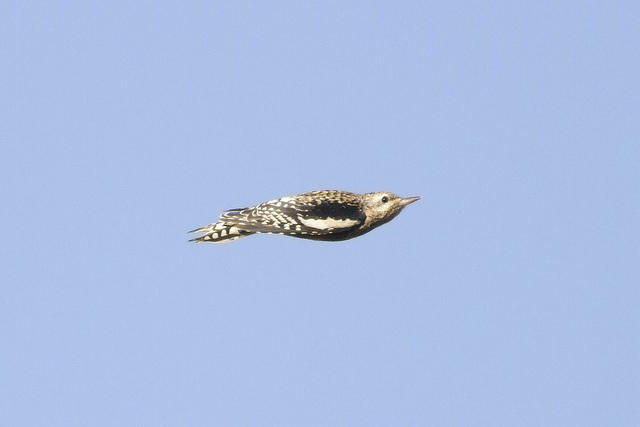In this detailed close-up photograph, a bird is captured mid-flight against a clear, light blue sky, devoid of any clouds. The bird is gliding horizontally with its beak pointed to the right and tail feathers extending towards the left. Its wings are tucked in closely along its sides, giving it a streamlined posture as if descending or increasing speed.

The bird has a striking appearance with intricate coloring and patterns. Its head is predominantly tan with tiny black and white eyes, and it has a light brown, short beak. The bird's body showcases a mix of black, white, and brown shades, with the top being tan. The wings exhibit a beautiful combination of black, white, and yellow lines and spots, emphasizing a striped design that continues onto the tail feathers, which also feature a white stripe pattern.

Positioned centrally in the frame, this bird stands out vividly against the serene backdrop of the sky, embodying grace and swiftness in its flight.